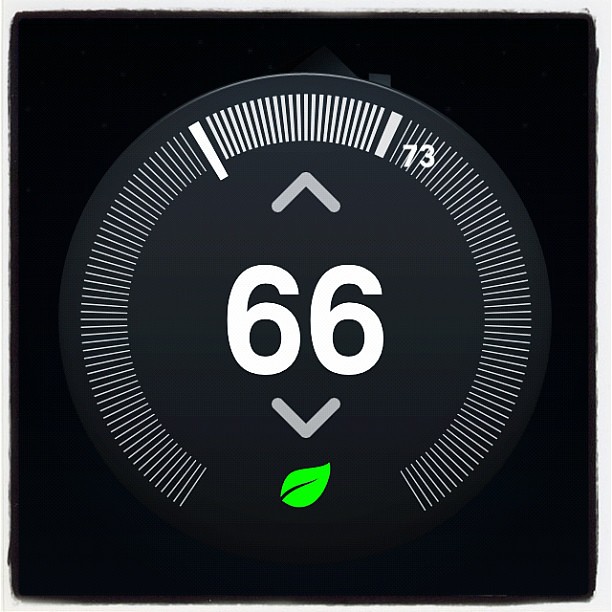A close-up image of a modern digital thermostat, currently set to 66 degrees Fahrenheit. The thermostat features two adjustment arrows, allowing the temperature to be increased or decreased. Below the temperature display, a green leaf icon is visible, often indicating eco-friendly settings. Additionally, a white bar on the display shows the temperature range, with the maximum limit at 73 degrees Fahrenheit. The midpoint of the bar appears to be around 66 degrees, although the minimum value is not indicated.